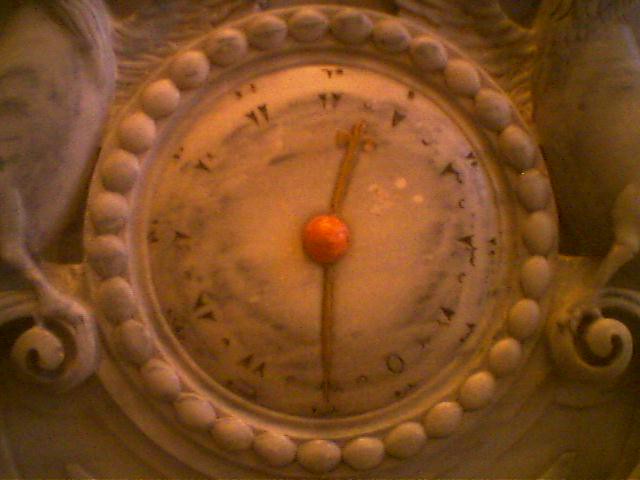This detailed close-up photograph captures a grainy image of a cream-colored, round stone clock, which is an integral part of a larger stone sculpture. The clock face, embedded with intricate black veins, suggests that the material may either be marble or a similarly veined stone. Surrounding the clock are additional stone carvings, seamlessly integrated into the same segment of stone, highlighting the cohesive nature of the sculpture.

Encircling the clock face, meticulously carved beads add a layer of ornate detail. The time is indicated by minute and hour hands, crafted from what appears to be gold, radiating a subtle elegance. Securing the hands at their center is a bolt of an orangish-pink hue, adding a touch of contrasting color to the predominantly cream and gold palette. 

Rather than traditional numerals, the hours are marked by unique symbols, primarily composed of single or double triangles, offering a distinctive and artistic alternative to conventional clock designs. The combination of the clock’s craftsmanship with the natural beauty of the stone creates a visually captivating and timeless piece of art.